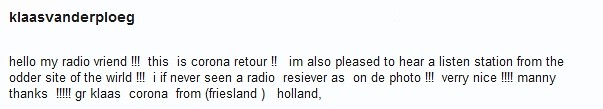The image appears to be a screenshot or a small photo of a text box displayed on a computer screen. The background of the image has a bluish-white tint. At the very top, in bold black text, are the words "KLAAS VANDER PLOEG." Below this, there is white text in a standard font that reads: "Hello, my radio friend!!! This is Corona Retour!! I’m also pleased to hear a listen station from the other side of the world!!! If never seen a radio receiver as on the photo!!! Very nice!!!! Many thanks!!!!! Klass Corona from Friesland, Holland." The message, written with several enthusiastic exclamation marks, appears to be a greeting or communication expressing joy at connecting with a radio station from a distant part of the world. The text also indicates that the sender hails from Friesland, Holland.